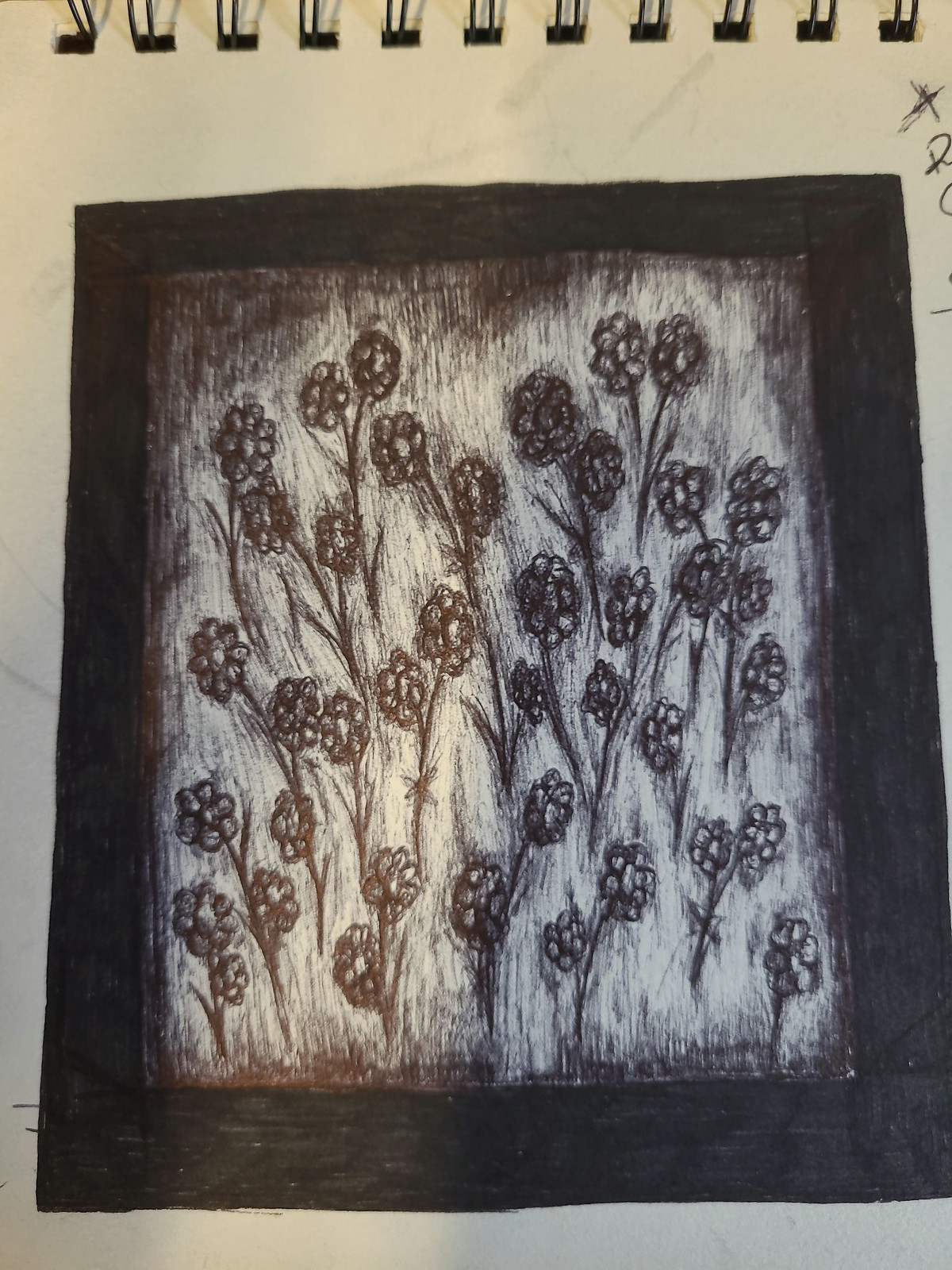The artwork in question is framed in a sophisticated black frame positioned in a portrait orientation. It features a masterful black and white drawing, created with what appears to be either charcoal or black ink. The composition is predominantly filled with an extensive arrangement of meticulously detailed flowers, each emanating from noticeably sturdy stems. Every stem supports a pair of flowers, and each flower distinctly displays six finely-crafted petals. The entire canvas is adorned with these floral elements, leaving no blank spaces. The artist's adept use of shading and intricate strokes not only accentuates the flower stems but also brings a textured, almost tangible depth to the background, enhancing the overall visual impact of this monochromatic masterpiece.